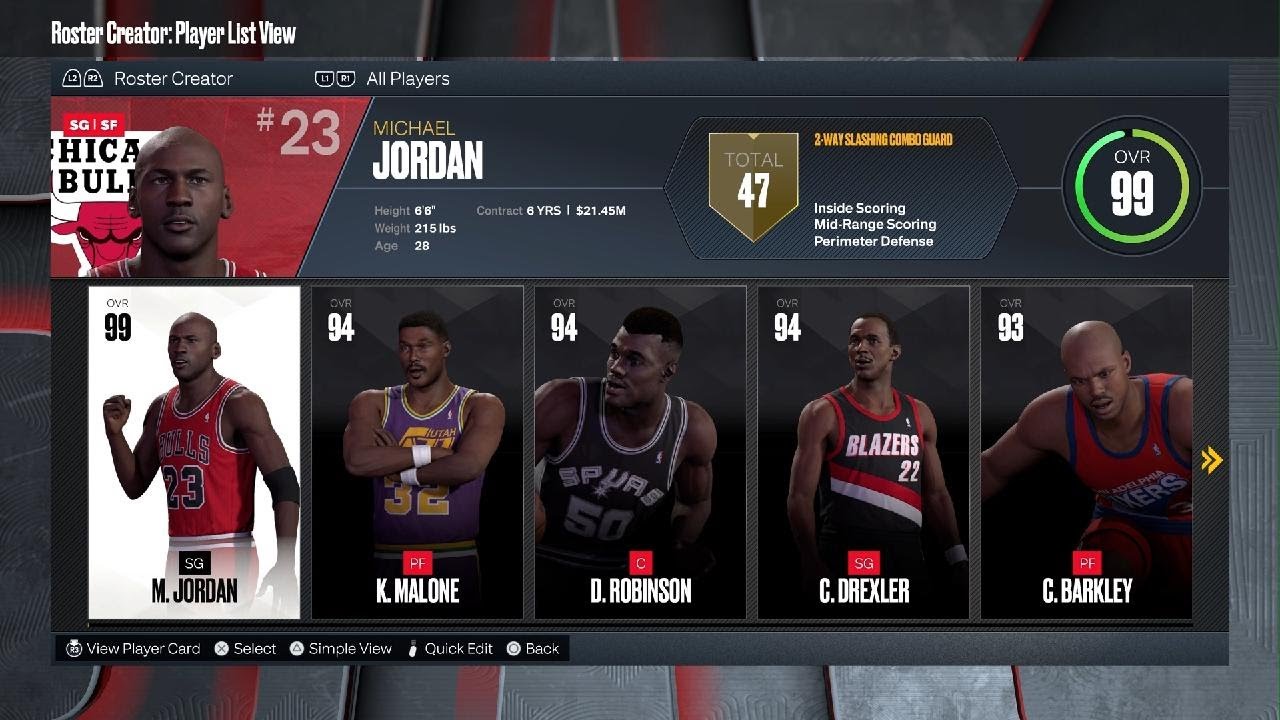Screenshot of a Video Game Interface: Roster Creator Playlist View

This detailed image is a screenshot from a video game, showcasing a menu titled "Roster Creator: Playlist View" in distinct white text. The background features an intricate pattern of black, gray, and red shades. 

At the top display, the game commands "L2/R2 - Roster Creator" and "L1/R1 - All Players" are listed in white, with "Roster Creator" and "All Players" terms capitalized. Below this, the screen presents a detailed player profile set against a black backdrop.

Central to the image is the graphic of a player depicted from the neck up, donning the Chicago Bulls' red uniform, with the number 23 prominently displayed. This is none other than the legendary Michael Jordan. His name is highlighted uniquely: "Michael" in vivid yellow text and "Jordan" in a metallic gold resembling shades of Las Vegas hues. "JORDAN" is further emphasized in bold white capital letters.

The profile continues with Jordan's essential stats: height, weight, age, contract details, and total earnings. His performance metrics outlined include categories such as inside scoring, mid-range scoring, perimeter defense, and his position as a three-way slashing combo guard. Notably, his overall rating (OVR) is impressive at 99, visually encircled by a striking green, though the circle is incomplete.

Additionally, five other player options are subtly indicated towards the bottom of the screen, with the prompt "Reload" signaling an update or refresh option within the game.